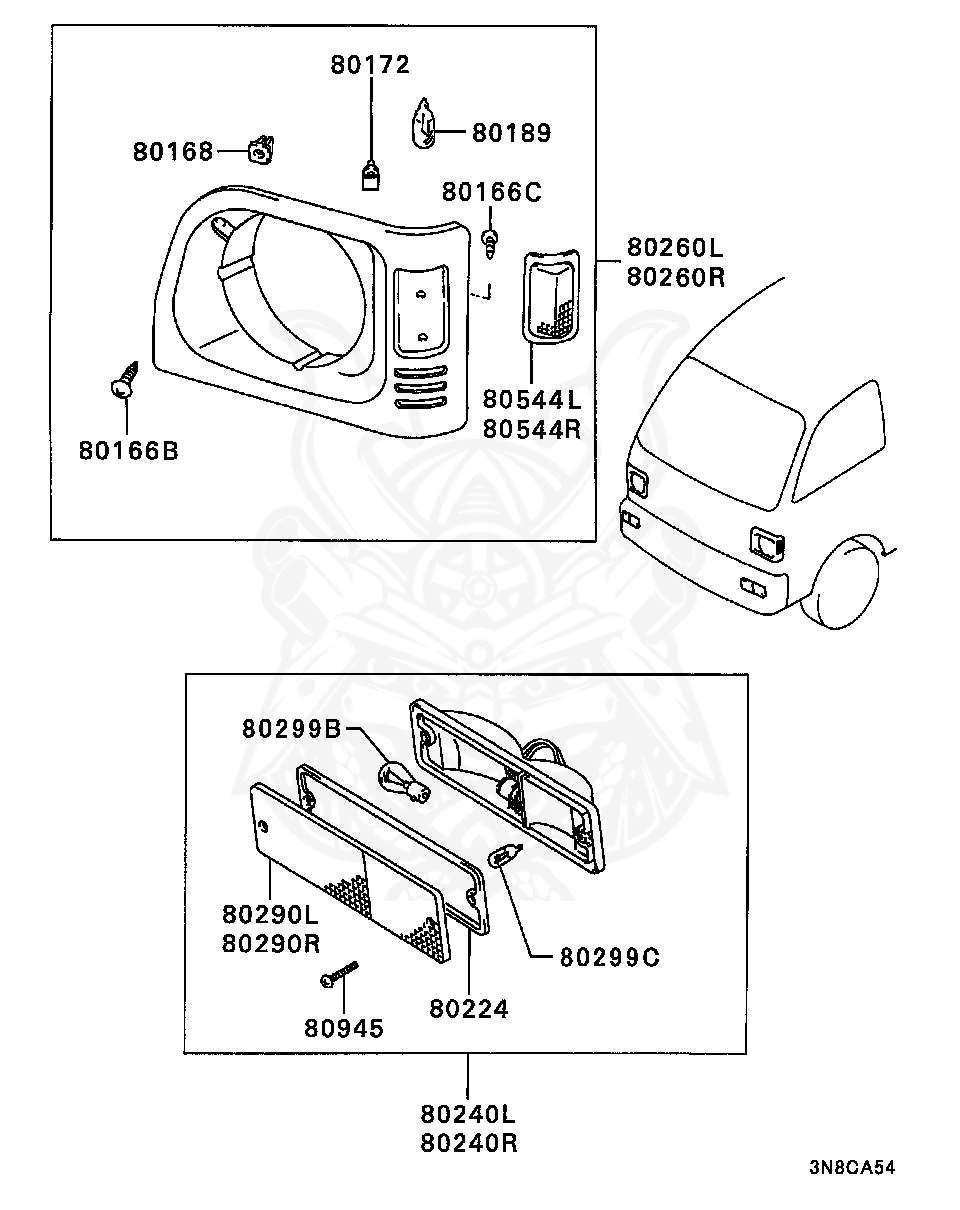This black and white schematic diagram elegantly lays out two critical components of a van, believed to be the front headlight and front reflector. The upper left box meticulously details the headlight, enumerating various parts with specific numbers like 80168, 80172, 80189, and 80544L/R, indicating items as small as screws and light bulbs. Below, a second boxed area delineates the front reflector, also thoroughly labeled with numbers such as 80299B, 80290L/R, and 80224, facilitating precise part identification and ordering. The diagram is overlaid with a watermark of a samurai face, adding a distinctive flair. To the right, a simplified sketch of the van front is partially visible, featuring the front window, side window, and a wheel, tying the components to their physical locations on the vehicle. In the lower right corner, the text "3N8CA54" appears, which could be a page or section indicator from a specialized manual.